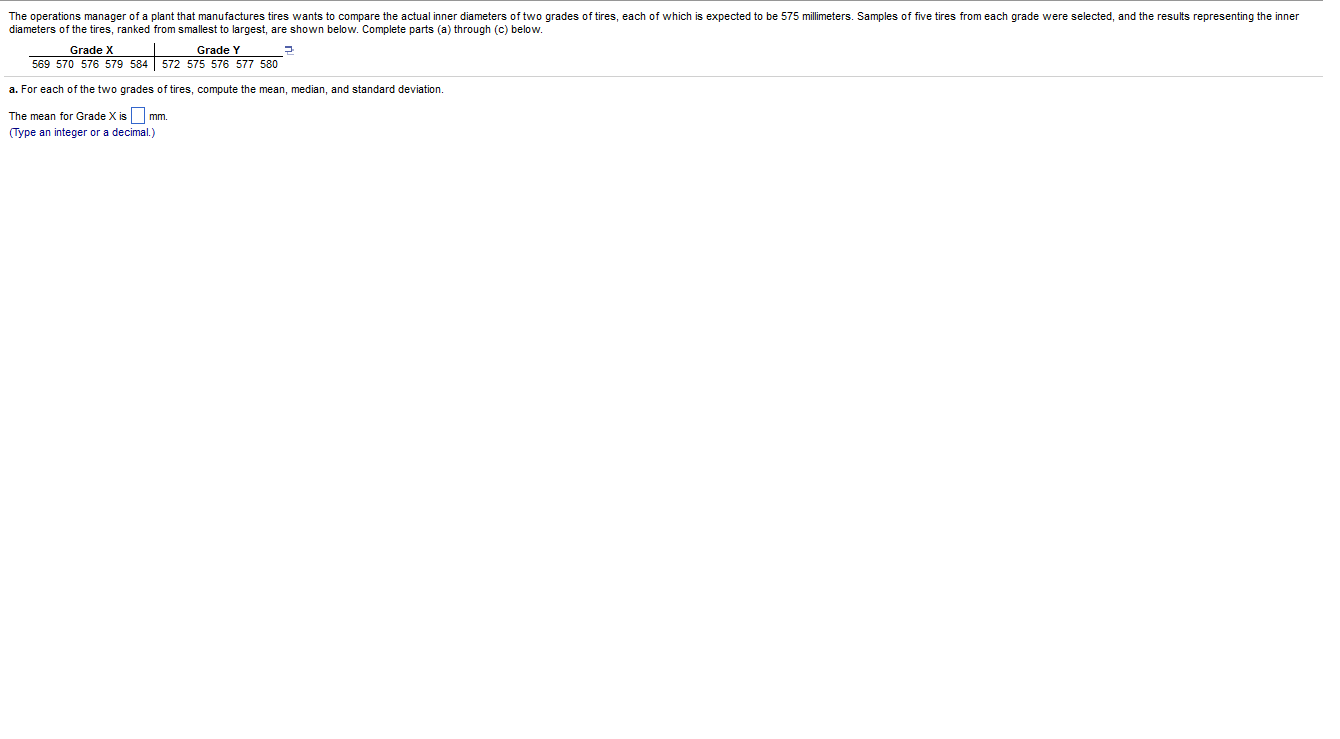The image contains a detailed comparison of the inner diameters of two grades of tires, each expected to be 575mm. The study measures the actual inner diameters for both grades. The data for Grade X are as follows: 569mm, 570mm, 576mm, 579mm, and 584mm. For Grade Y, the inner diameters measured are 572mm, 575mm, 576mm, 577mm, and 580mm. The caption also prompts the computation of the mean, median, and standard deviation for each grade. Additionally, there is mention of completing parts A through C related to the statistical analysis of the tire measurements. The background shows text instructions for the analysis process, emphasizing the need to get accurate figures of central tendency and variability for each tire grade. The overall context implies a focus on evaluating the manufacturing accuracy of the tire diameters compared to the expected standard.